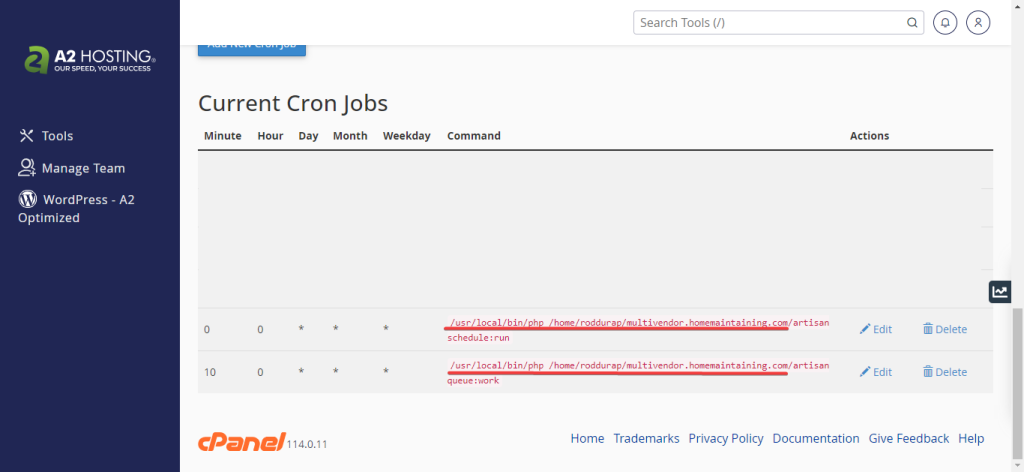The image is a screenshot of a website with a white background. Along the left side, there is a navy-colored column. In the upper left corner of this column, there is a green logo depicting the letter "A." Adjacent to the logo, white text reads "A2 Hosting, Your Speed, Your Success." Below this heading, there are several menu options listed: "Tools," "Page Team," "WordPress," and "A2 Optimized."

To the right of this column, the background is white. In the upper right corner, there is a search bar containing the text "Search Tools." Below this, the section is titled "Current Cron Jobs," with the words "Minute," "Hour," "Day," "Month," "Weekday," "Command," and "Actions" listed underneath.

Directly below this section, there is a gray area featuring underlined red text that presumably indicates file locations. Next to these file locations, there are blue "Edit" and "Delete" buttons. 

At the bottom of the image, an orange label reads "C Panel," followed by links in blue text to "Home," "Trademarks," "Privacy Policy," "Documentation," "Give Feedback," and "Help."